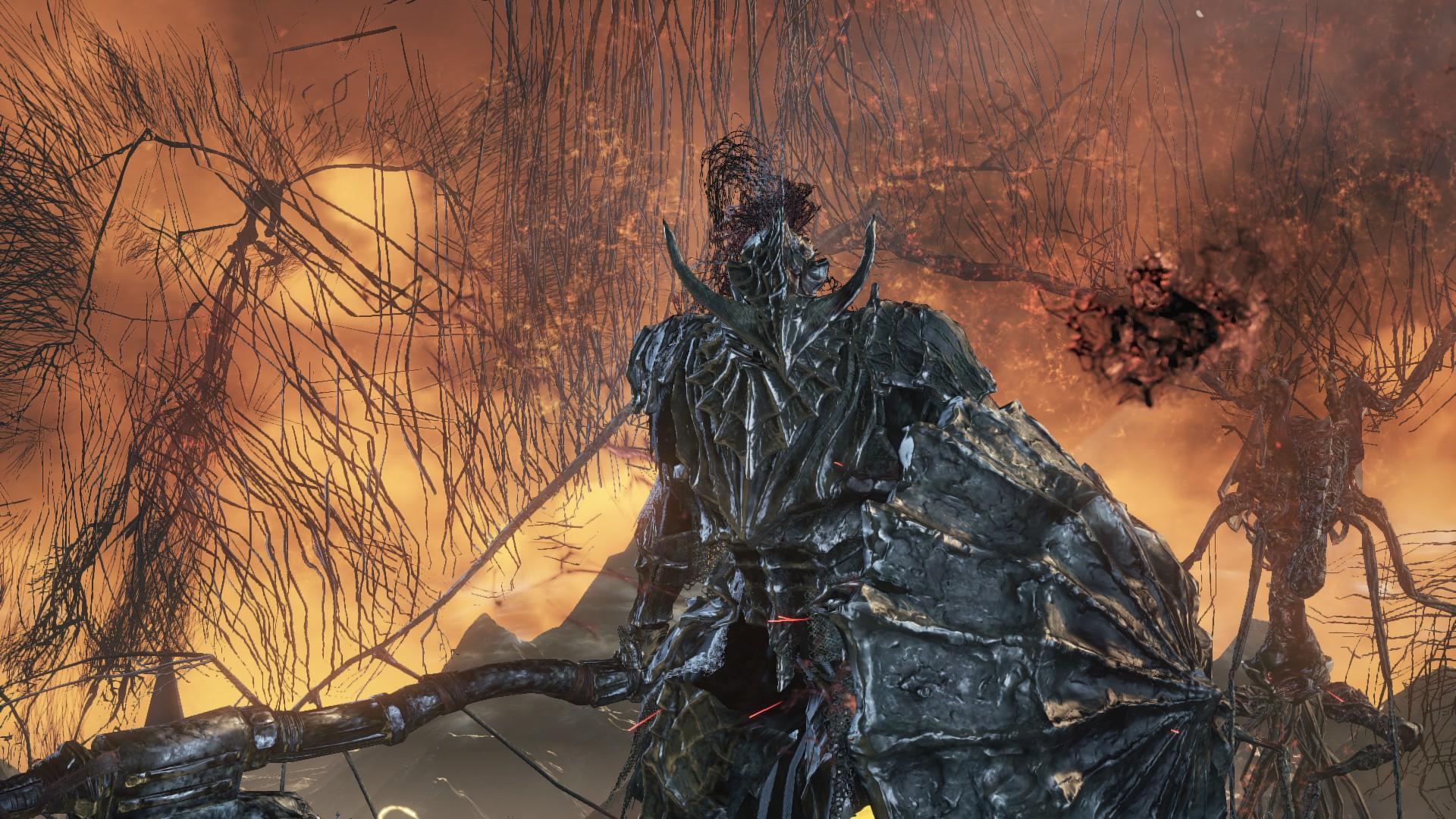In this vivid illustration, we see a central armored character set against a fiery orange background interspersed with gray smoke and vein-like, dark, tree-like objects that span almost the entirety of the backdrop. The figure is clad in matte, metallic, very dark gray armor, detailed with an intricate spiderweb pattern around the collar. The imposing helmet features two long, pointed horns jutting out from the front. The armor itself has a ridged texture, resembling cast iron. The character wields a long, twisted gray weapon with a large, mechanized end, and bears a large, rounded shield with prominent gray ribs, reminiscent of an inverted umbrella. The eerie setting is completed by the presence of dead, dried-up, thin, grassy-looking trees, and mysterious, almost organic, metallic forms. The scene presents a striking, science-fiction aesthetic that evokes the cover of a book or a still from a movie.